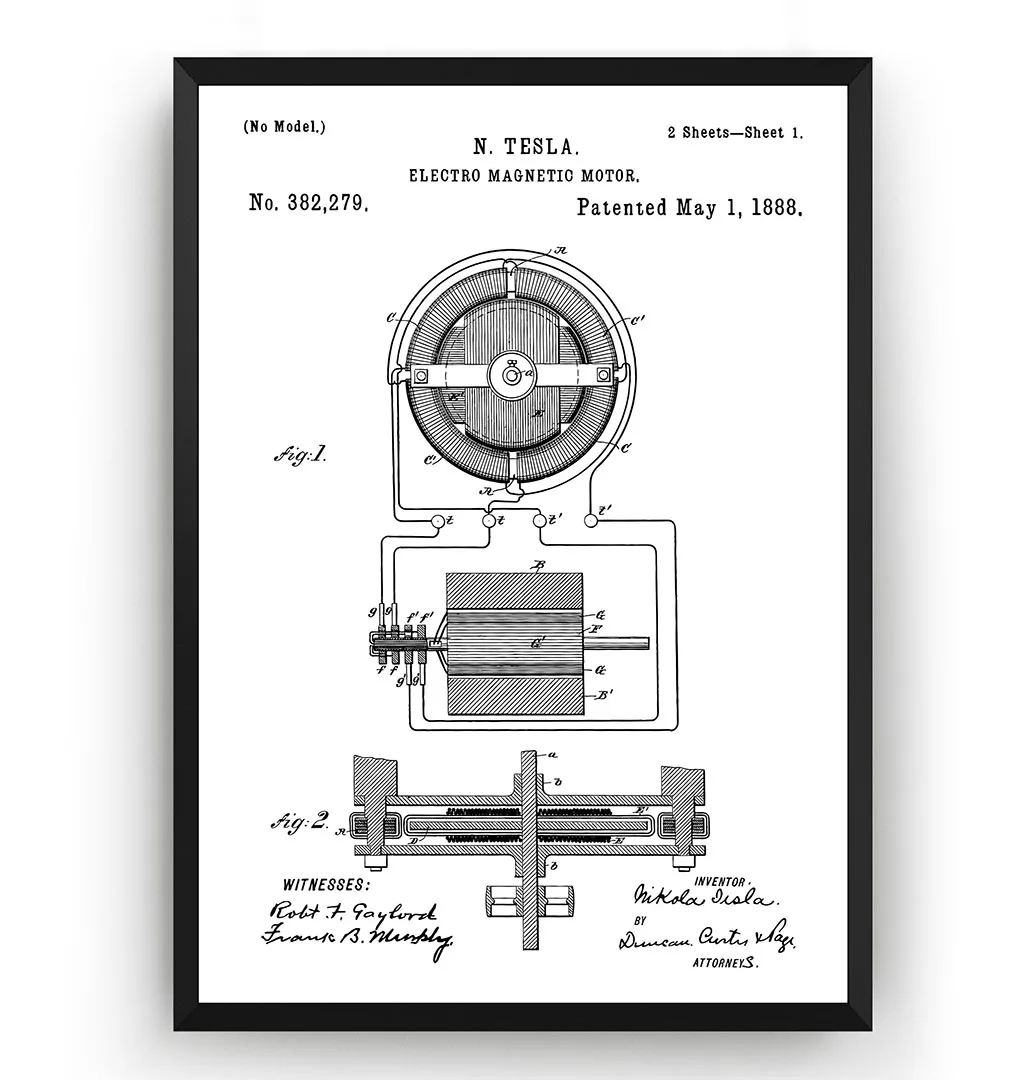This image displays a detailed black and white diagram of a Tesla magnetic motor, meticulously framed in a thin, simple black frame and mounted against an off-white light gray background. The prominently titled "N. Tesla Electromagnetic Motor, number 382,279, patented May 1st, 1888" occupies the upper center of the diagram. The black ink on white paper sketch illustrates the intricate components of the motor. 

In the upper section labeled "Figure 1," the diagram depicts a circular section of the motor with wires extending from the perimeter downwards, connecting to a square section that houses a horizontal bar. Below it, another diagram labeled "Figure 2" presumably shows an alternative angle of the motor, revealing a T-shaped configuration with multiple layers on its upper horizontal bar. Additionally, the document contains significant textual elements, including "No model, two sheets, sheet one," and mentions witnesses whose signatures are slightly readable. The signature of the inventor, Nikola Tesla, is featured alongside an attorney's name, which remains indecipherable. This framed piece is both a technical blueprint and an artifact of historical significance, showcasing the meticulous engineering prowess of Nikola Tesla.